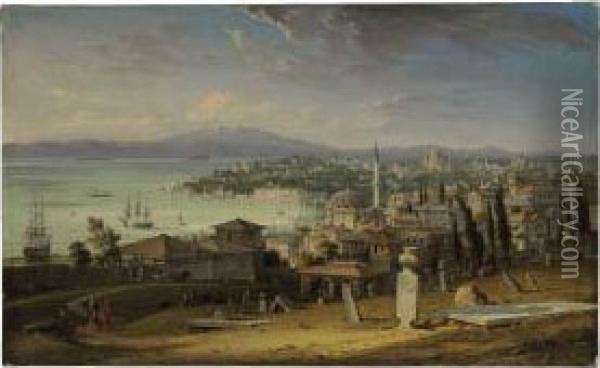This image, attributed to niceartgallery.com with text displayed vertically on the right-hand side, features an out-of-focus painting rendered in blues, grays, and browns. The scene depicts a historic port city bustling with activity. Dominated by tall towers and rounded domes, the city's skyline is intricate and expansive. To the left, a large body of water, possibly a lagoon or ocean, is dotted with both large ships and smaller sailboats. The sky above is filled with clouds, white in the distance and darkening as they approach the viewer. In the foreground, there appears to be a cemetery with various tombstones. Surrounding the city is a mix of sandy roads, greenery, and possibly a mountainous backdrop, enhancing the landscape's depth. Despite the overall blurriness of the image, the historic and serene essence of the painting is palpable.